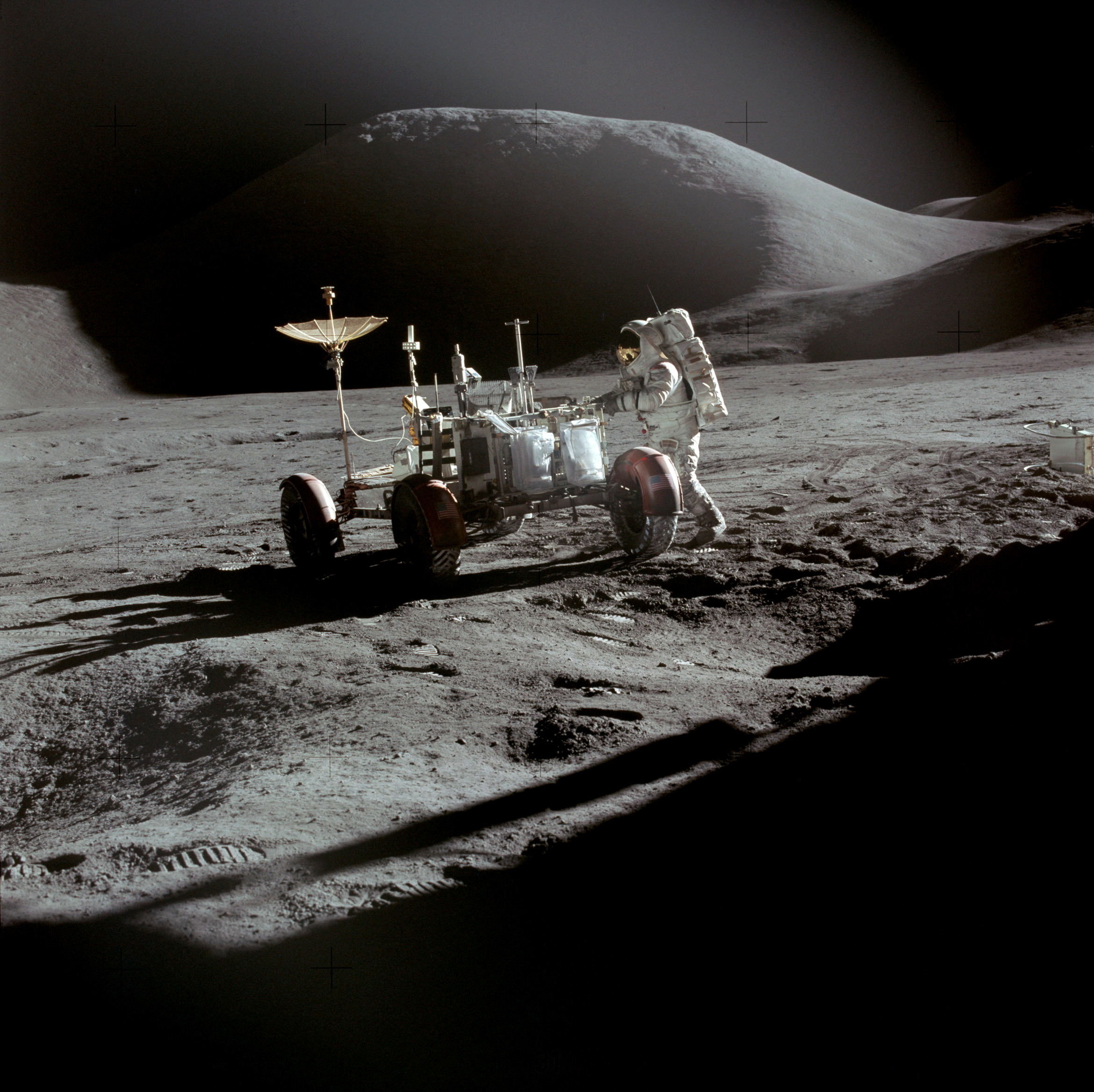This color photograph, likely generated by AI, depicts a surreal lunar scene. At the center of the composition, an astronaut stands beside a peculiar lunar vehicle. The vehicle is an assemblage of pipes and parts, seemingly incomplete, with a strange symbol or possibly an inverted satellite dish attached to its left side.

The background features a stark black sky, enhancing the otherworldly atmosphere. A hill is discernible in the distance, although it fades into the sky due to shadow, creating an eerie and continuous horizon. Adding to the surrealism, a black cross-like structure is visible towards the right side of the hill, contributing to the sense of an optical illusion.

Shadows also obscure the lower right corner of the image, amplifying the mysterious and disjointed elements of the scene. The overall composition combines the uncanny presence of the cross, the enigmatic vehicle, and the obscure landscape, leading to a somewhat confusing and poorly executed visual illusion.